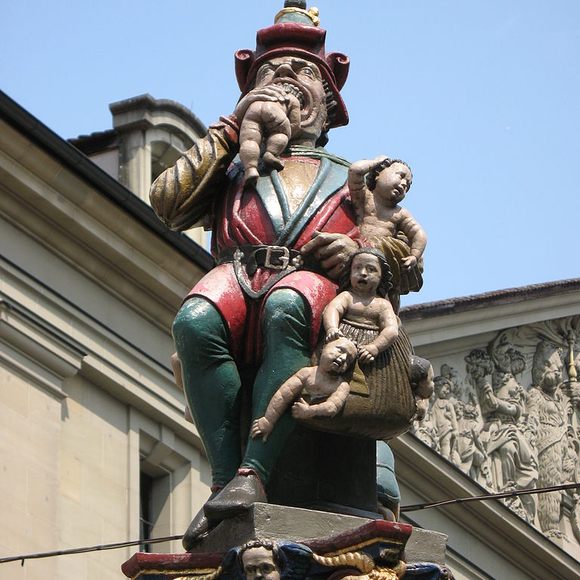The image features a detailed statue of a grotesque, goblin-like figure as the focal point. The figure has a somewhat human-looking face with large eyes and furrowed eyebrows, and is depicted wearing a red hat adorned with gold detailing. He is dressed in a red jacket with a blue collar, a black belt, green pants, and black shoes. In his right hand, he grasps a naked baby, whose head is partially in his mouth, showcasing black teeth. In his left arm, the figure tightly cradles three other young children, their fearful expressions evident as they cling to him. The statue is perched upon a gray pedestal that shows visible detailing of a cherub at the bottom. Behind the statue, there is a carved frieze depicting a classical illustration, and to the left, the roof and window of another historic-looking building are visible.